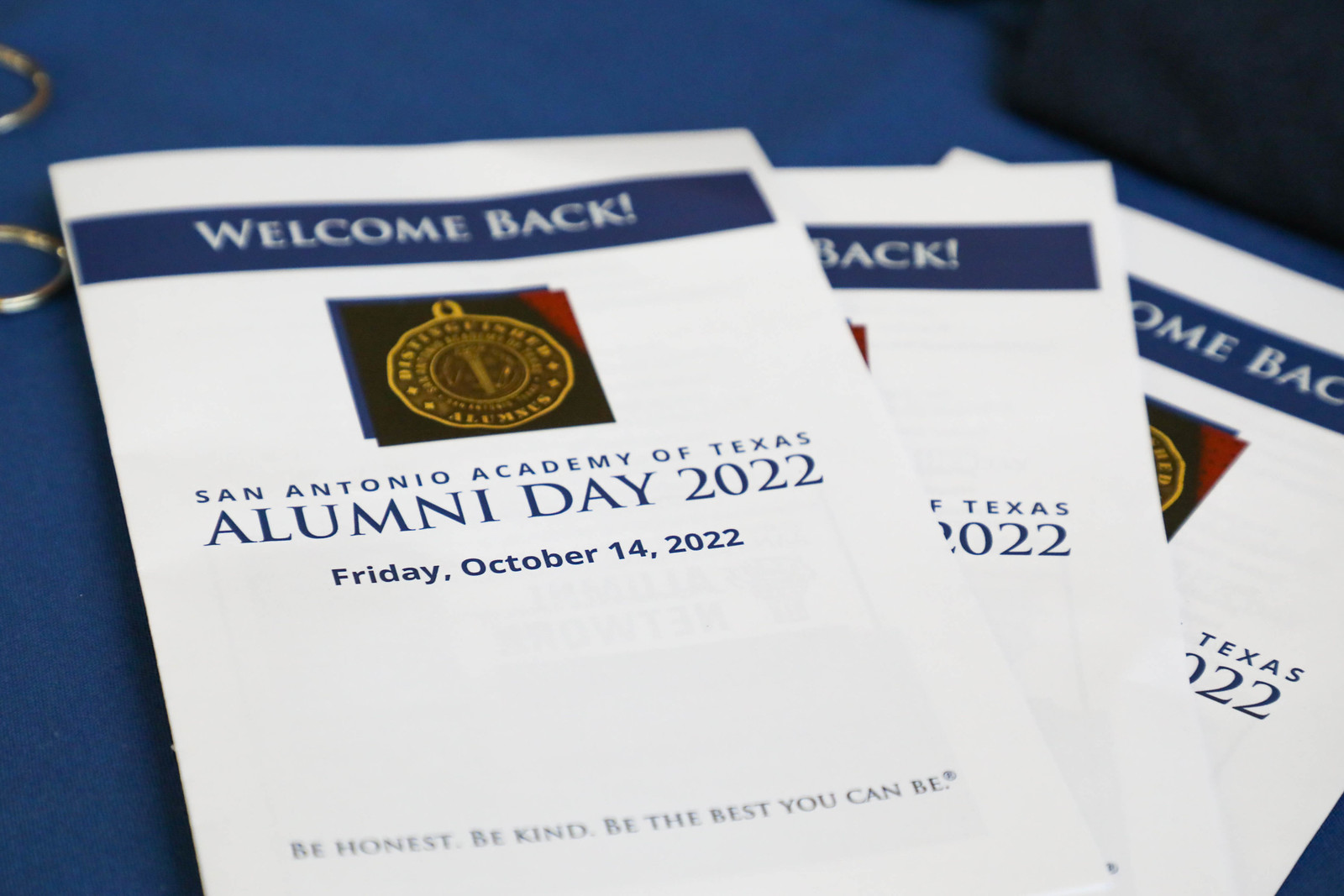The image captures a professional photograph of three brochures arranged on a blue table. The brochures, which are primarily white, also feature a blue horizontal stripe at the top reading "Welcome Back!" in white text. Below this, there is a small square with a black background showcasing a gold medallion, likely a logo for the San Antonio Academy of Texas. The text below the medallion, in blue font, reads "San Antonio Academy of Texas," followed by "Alumni Day 2022, Friday, October 14, 2022." Towards the bottom of the brochures, in gray text, are the words "Be honest, be kind, be the best you can be." The pamphlets are slightly stacked with the main one fully visible in the center left, and the others partially visible beneath it. Additionally, there is a subtle presence of silver rings, possibly from a binder, at the top left corner of the image.